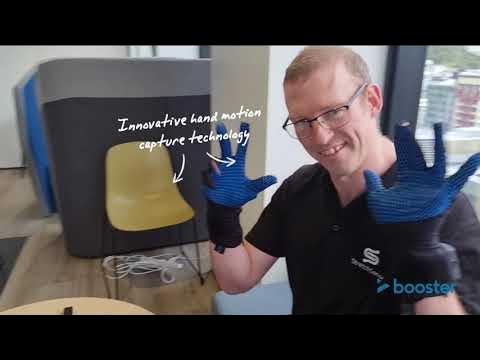The image appears to be an advertisement featuring a smiling Caucasian man with short, close-cropped brown hair and glasses, seated in an office setting. He is wearing a black short-sleeve shirt with indiscernible white lettering on it, along with distinctive black and blue gloves, with blue palms and black wrists. The man holds his hands up in front of him, palms facing the viewer and fingers spread out. To his left, there's a gray wall with a bright yellow chair placed against it; the chair has white cords trailing from its bottom. Next to the yellow chair, white text reads "Innovative Hand Motion Capture Technology." On the bottom right corner of the photo, the word "booster" is written in lowercase blue letters. The scene is framed by thin black strips at the top and bottom, and a window is visible behind the man, contributing to the office ambiance. A light wood laminate floor and a small strip of a tan table are also visible in the background, adding more context to the setting.